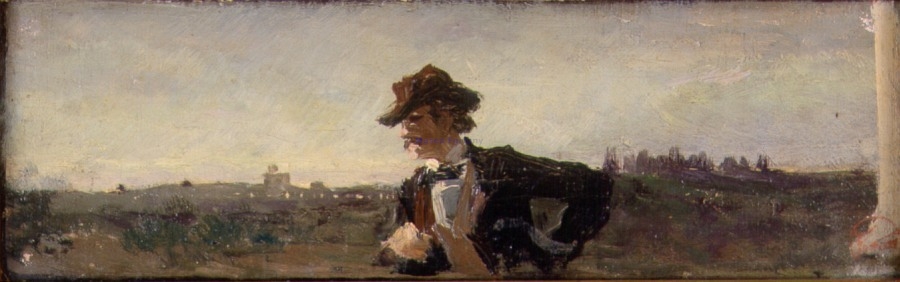The image is a horizontally-oriented painting that exudes a historical charm, likely from the 19th century or early 20th century. At its center stands a man dressed in vintage attire, characterized by a brown hat, a green coat paired with a matching bow tie, a white shirt, and a vest. He sports a mustache and has shoulder-length wavy brown hair. The man is depicted walking from right to left, with his hand on his hip and the other hand gesturing in front of him, creating a sense of movement. His attire and posture suggest a confident, almost leisurely stroll.

Behind him stretches an unfocused, impressionistic backdrop of a town or cityscape, possibly reminiscent of Paris. The horizon glows brighter with soft, unfocused clouds, transitioning into darker, overcast skies as they ascend towards the top of the painting. To the right of the man, there's a white column that could either belong to a Roman-style pillar or the porch of a house, hinting at architectural elements supporting an upper structure.

In the distance, a small town is discernible through a prairie-like field, further enhancing the nostalgic and serene atmosphere of the painting. The entire composition, though slightly blurry and lacking in fine details, evokes a sense of timelessness and captures a quiet moment in a bygone era.